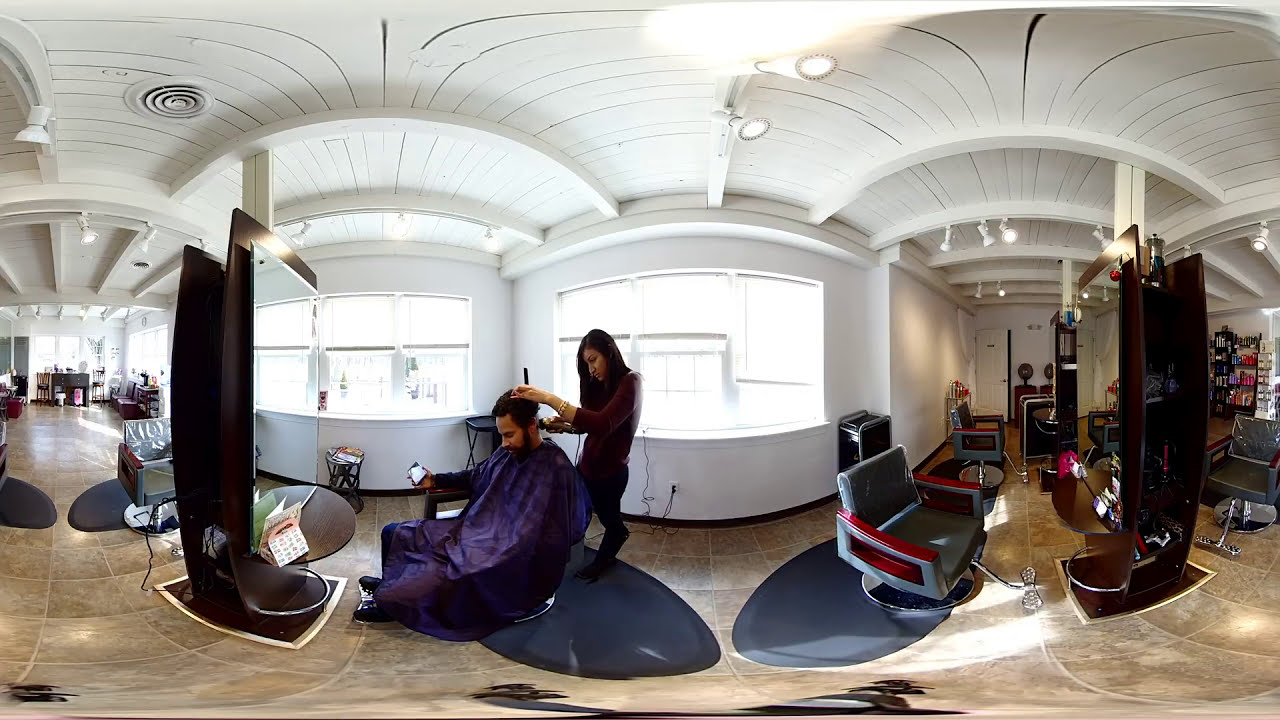This image depicts a spacious, modern, and upscale hair salon with a sophisticated design, likely captured with a wide-angle lens to emphasize the extensive layout. The salon features multiple workstations, although only one customer is currently visible. In the center of the image, a bearded man draped in a purple wrap is seated in a beautician's chair, facing left. A woman with long hair, dressed in dark clothing, is meticulously trimming his hair, using a comb in her left hand and a razor in her right. The floor beneath the chairs is adorned with attractive old rugs, and each beautician's station includes rounded tables equipped with various supplies.

The salon is well lit with numerous ceiling lights, enhancing its clean and modern aesthetic. The ceiling itself showcases beautiful arched decorations. The area on the right side of the image extends back to a wall that displays shelves stocked with beauty supplies such as hairsprays, shampoos, and conditioners. Further back, a few seated hair dryers are visible. The salon gives an impression of meticulous organization, with no visible clutter or hair on the floor, suggesting a high level of cleanliness and sophistication. The predominantly white walls and the abundance of windows contribute to a bright and inviting atmosphere. While no text is visible in the picture, the overall ambiance suggests an exclusive and costly service environment.